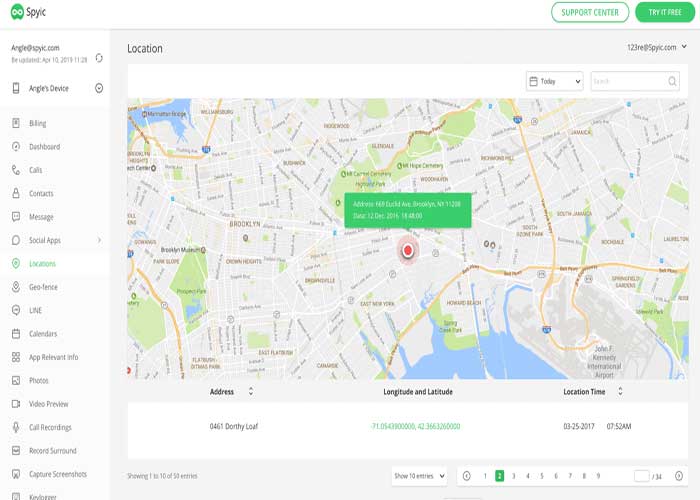The image displays a website on a computer screen, focusing on a map interface. The website features a white background with black text, while the map itself has a beige background accented with black lettering for various locations. At the top left corner of the screen, there is an inscription that appears to read "SPYIC," accompanied by a small, round green icon featuring an infinity symbol. 

To the right, there is clickable green text that says "Support Center," partially obscured by a picture box in front of it. The text "Try it free" is visible and evidently part of a marketing call to action. The left sidebar hosts a vertical menu that includes categories like "Argyle SPYIC.com" and "angle SPYIC.com," though these lists are somewhat blurry and hard to decipher. The sidebar continues with options like "Dashboard," "Calls," "Contacts," "Messages," "Social Apps," "Geofence," "Calendar," "Photos," "Call Recordings," "Video Preview," and "Record Captive Screenshots."

The central portion of the screen prominently displays the map, marked with a conspicuous red dot, likely indicating a specific location or target. The clarity of the image is not perfect, but near the bottom of the map, three fields provide details under the headings "Address" (with navigational arrows), "Longitude and Latitude," and "Location Time," indicating that this part of the website is used for tracking.

At the bottom of the screen is pagination that allows navigation between pages numbered 1 through 9, suggesting multiple sets of data or screenshots. An additional feature allows toggling the display to show 10 entries at a time. Underneath the address section, specific details such as the actual address, coordinates, and the timestamp (March 25, 2017) are visible. Overall, this website appears to be a tracking or monitoring platform, potentially a spying tool, designed to locate and log positions over time.